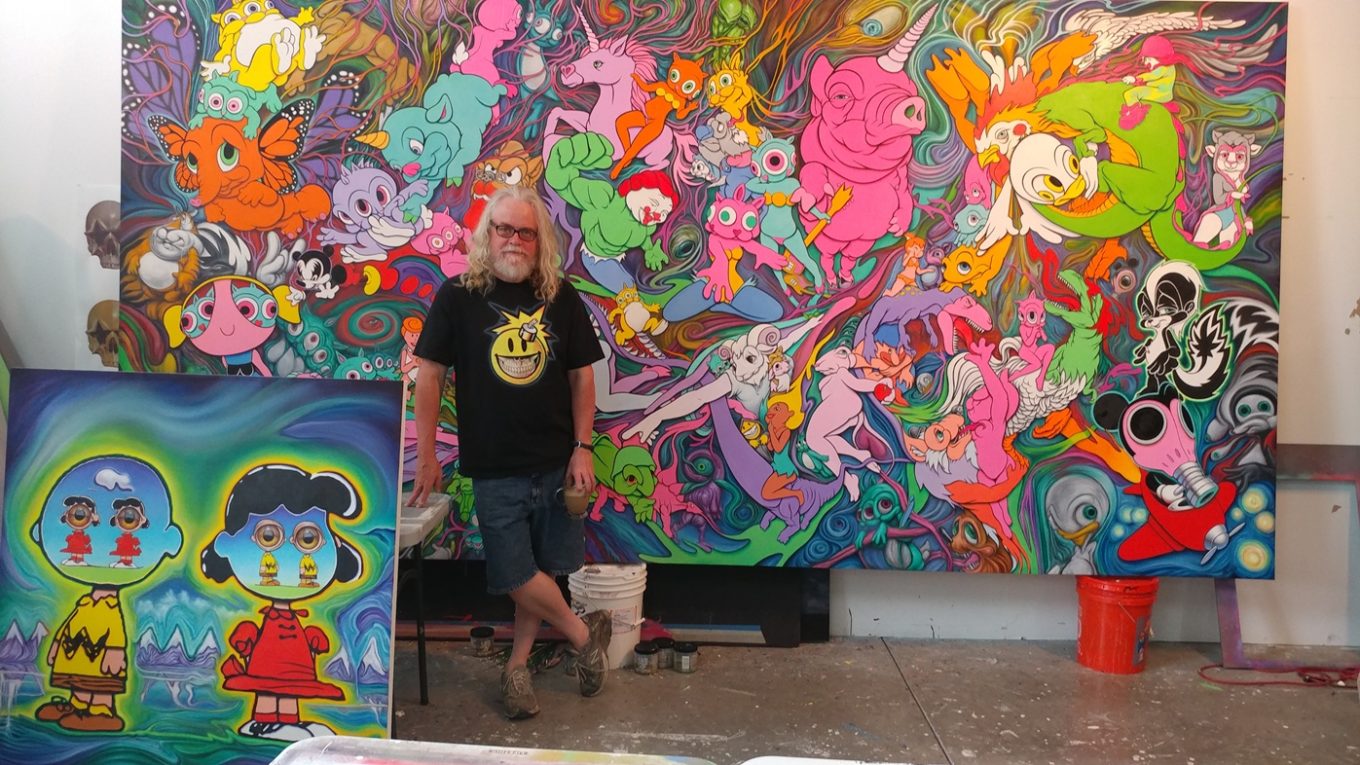A man with long gray hair, a full beard, and black-rimmed glasses stands on a concrete floor in front of a large, vibrant, and whimsical mural that nearly covers an entire white wall. The mural behind him showcases a variety of fantastical characters, including a unicorn, dragon, little girl, skunk, and a superhero with a clown face and ruby red hair. The colors in the mural are striking, featuring pinks, whites, yellows, lime greens, and more.

The mural appears to be supported by five-gallon buckets: one red bucket on the right and a white bucket in the center. To the left of this large mural, a smaller painting rests on the floor, leaning against a white table. This painting depicts an unusual version of Charlie Brown and Lucy where their eyes are replaced by each other's figures. Charlie Brown's eye features Lucy's entire body and vice versa. Both characters are drawn with vibrant colors, Lucy in her red dress and bobby socks and Charlie Brown in his yellow shirt with a black zigzag stripe.

The man, who faces the camera with a slight lean on his left leg and his right leg bent at the knee and crossed over, wears a black t-shirt with a large yellow smiley face displaying a toothy grin, along with jean shorts. He holds a cup in one hand and wears a watch on his left wrist, embodying a casual and approachable demeanor.